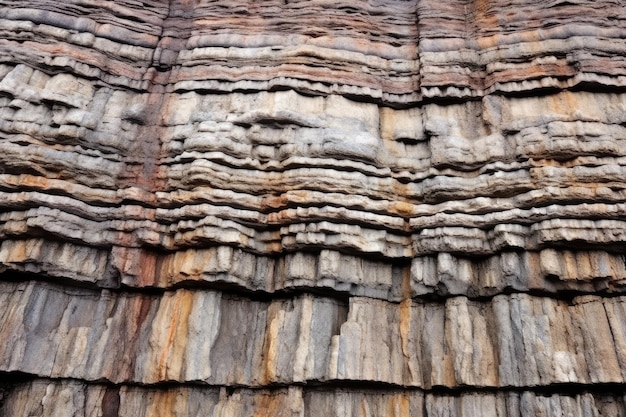The image is a horizontally aligned rectangular close-up of a wood-shingled roof with no borders or text. The layers of wood shingles, which are pressed together and aligned horizontally, span from the bottom to the top of the image. The shingles display a variety of colors, including medium brown, light brown, grayish brown, and dark brown, with white highlights suggesting reflections from sunlight. The shingles are more defined and broader at the bottom and gradually become smaller, forming overlapping patterns as they ascend. The top portion of the image is slightly blurry. The scene evokes an old wooden house, reminiscent of structures from the 1920s to 1940s, with the intricate texture of the wood showcasing both natural wear and the effects of aging.